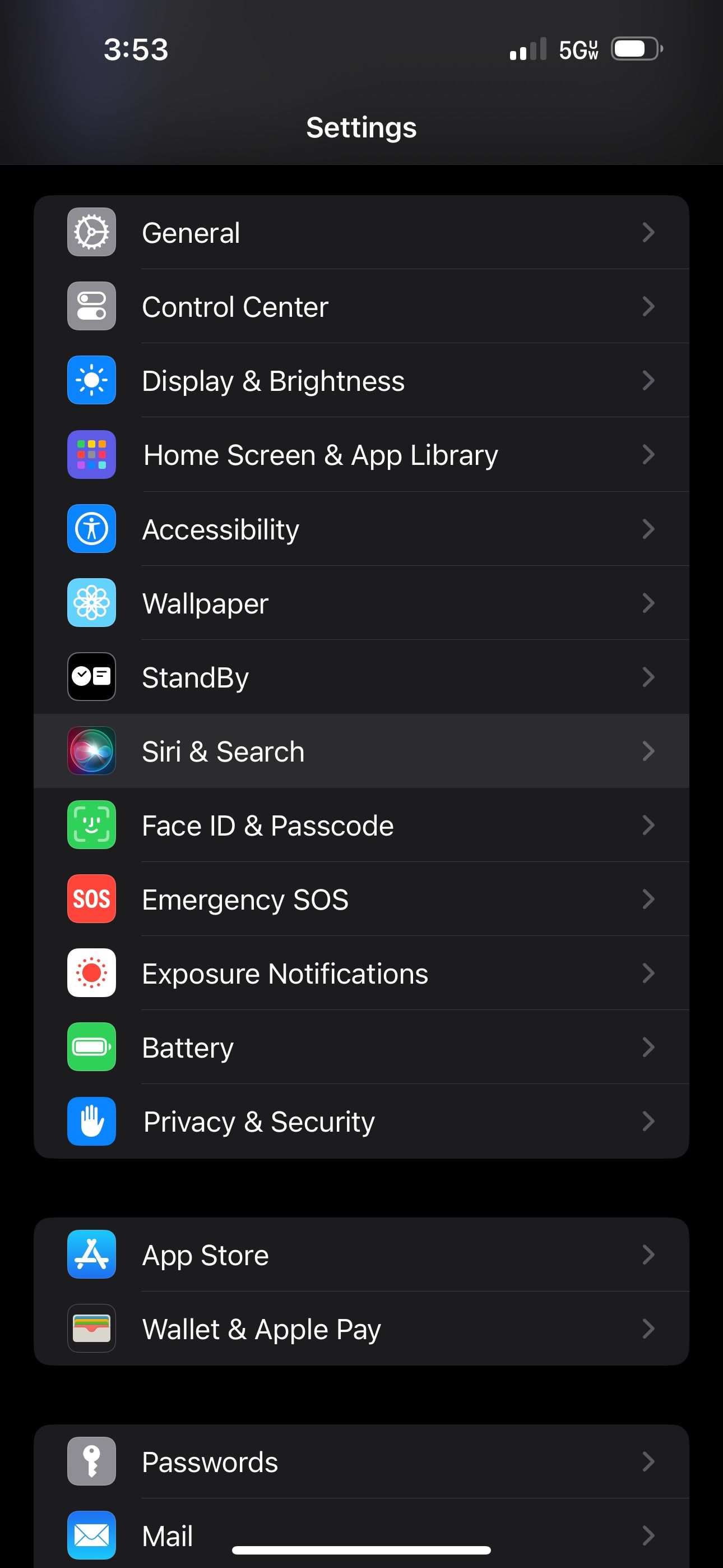The image features a screenshot from an iPhone, identifiable by its distinct iOS design and iconography. The screenshot displays the main page of the iPhone's Settings app, showcasing a comprehensive list of settings options. Visible settings include General, Control Center, Display & Brightness, Home Screen & App Library, Accessibility, Wallpaper, Standby, Siri & Search, Face ID & Passcode, Emergency SOS, Exposure Notifications, Battery, Privacy & Security, App Store, Wallet & Apple Pay, and Passwords & Mail. Although the full list extends beyond the screen, most options are visible due to the lengthy display. Notably, the "Siri & Search" setting is highlighted with a different background color, indicating that it has been selected.